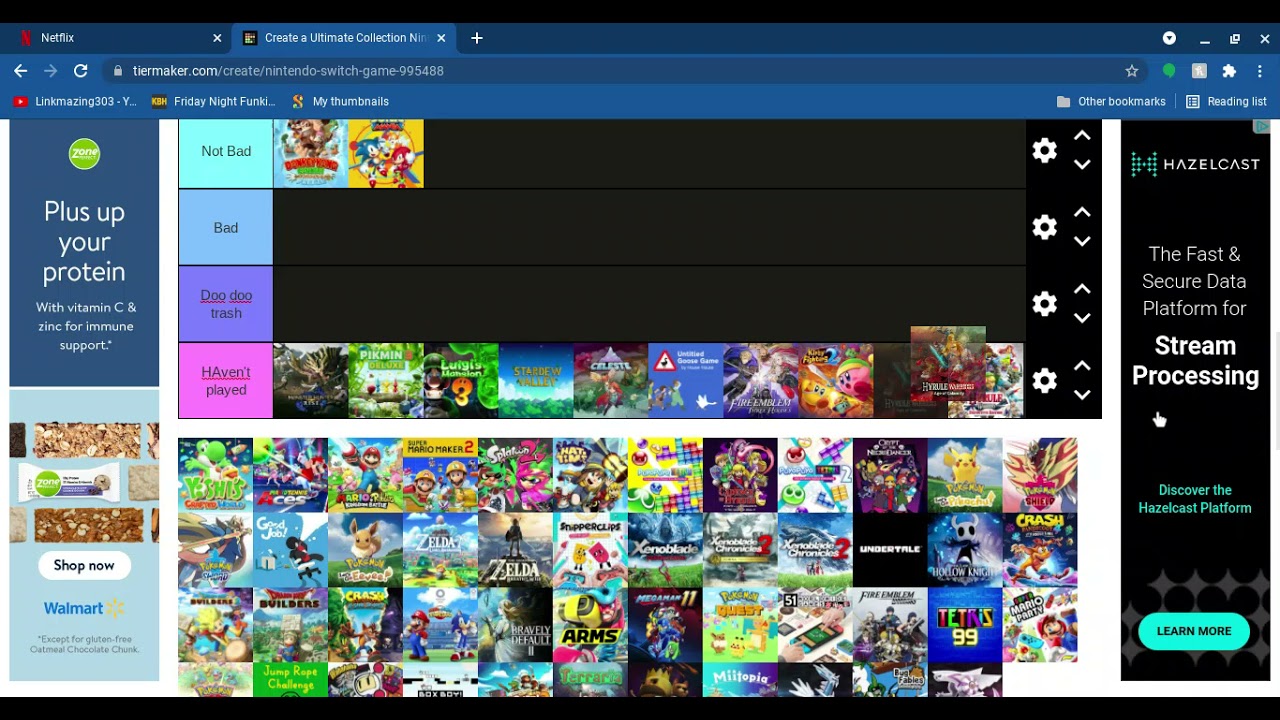The image depicts a website open in a browser window with two active tabs: "Netflix" and "Create an Ultimate Collection - Nintendo Switch Games." The visible, active tab is on a website named "tiermaker.com," specifically on a page for creating a Nintendo Switch game tier list (URL: tiermaker.com/create/nintendo-switch-game-995488).

On the left side of the screen, there are two advertisements. One reads, "Plus up your protein with vitamin C and zinc for immune support," and the other is a shopping ad from Walmart. 

The top section of the website features a black background with several filled-in boxes. The left sidebar appears to contain a rating system with the following categories: "Not Bad" (green), "Bad" (blue), "Doo-Doo Trash" (purple), and "Haven't Played" (pink). The titles "Not Bad" and "Bad" contain some items, though they are too blurry to identify. 

Under the "Haven't Played" category, there are 10 items listed. At the bottom of the screen, there is a large collection of different Nintendo Switch game icons. It appears that one game is in the process of being moved, as its icon is positioned slightly above the others. This interface indicates that users can drag and drop games into different categories to create their personalized tier list.